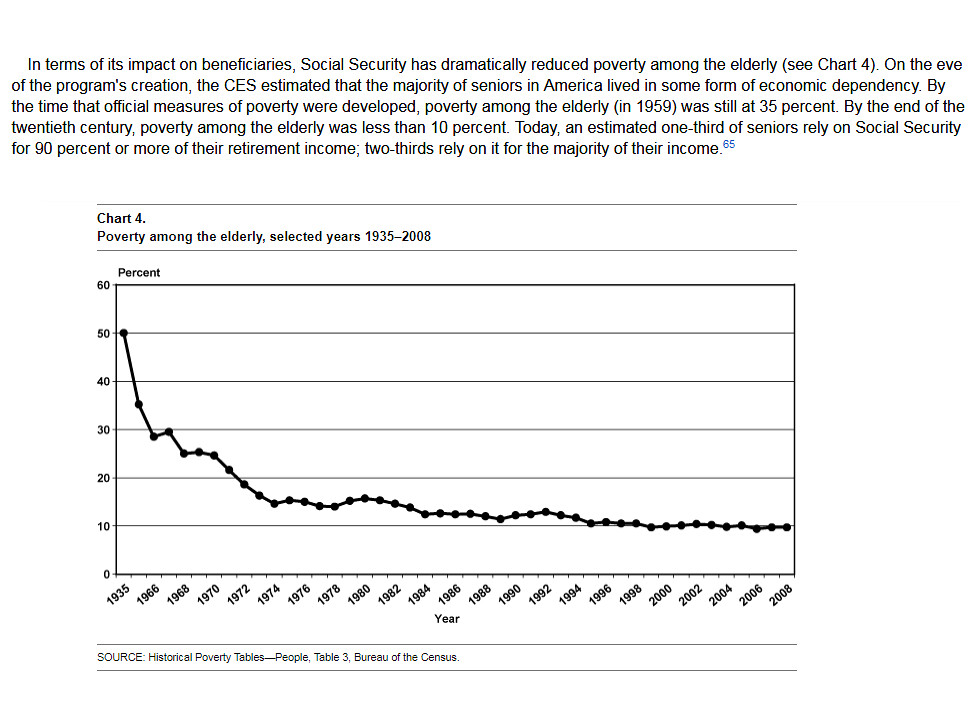The image displays a black and white line graph on a solid white background with a detailed paragraph of text above it. The black-font paragraph reads: "In terms of its impact on beneficiaries, Social Security has dramatically reduced poverty among the elderly, see Chart 4. On the eve of the program's creation, the CES estimated that the majority of seniors in America lived in some form of economic dependency. By the time the official measures of poverty were developed, poverty among the elderly in 1959 was still at 35%. By the end of the 20th century, poverty among the elderly was less than 10%. Today, an estimated one-third of seniors rely on Social Security for 90% or more of their retirement incomes. Two-thirds rely on it for the majority of their income." Below this text, the line graph titled "Chart 4: Poverty Among the Elderly, Selected Years 1935-2008" depicts poverty trends among the elderly over time. The vertical axis shows percentages ranging from 60% to 0%, while the horizontal axis spans from 1935 to 2008. The graph illustrates a significant decline in elderly poverty from around 50% in 1935 to below 10% by 2008. The source of the data is "Historical Poverty Tables - People Table 3, Bureau of the Census."